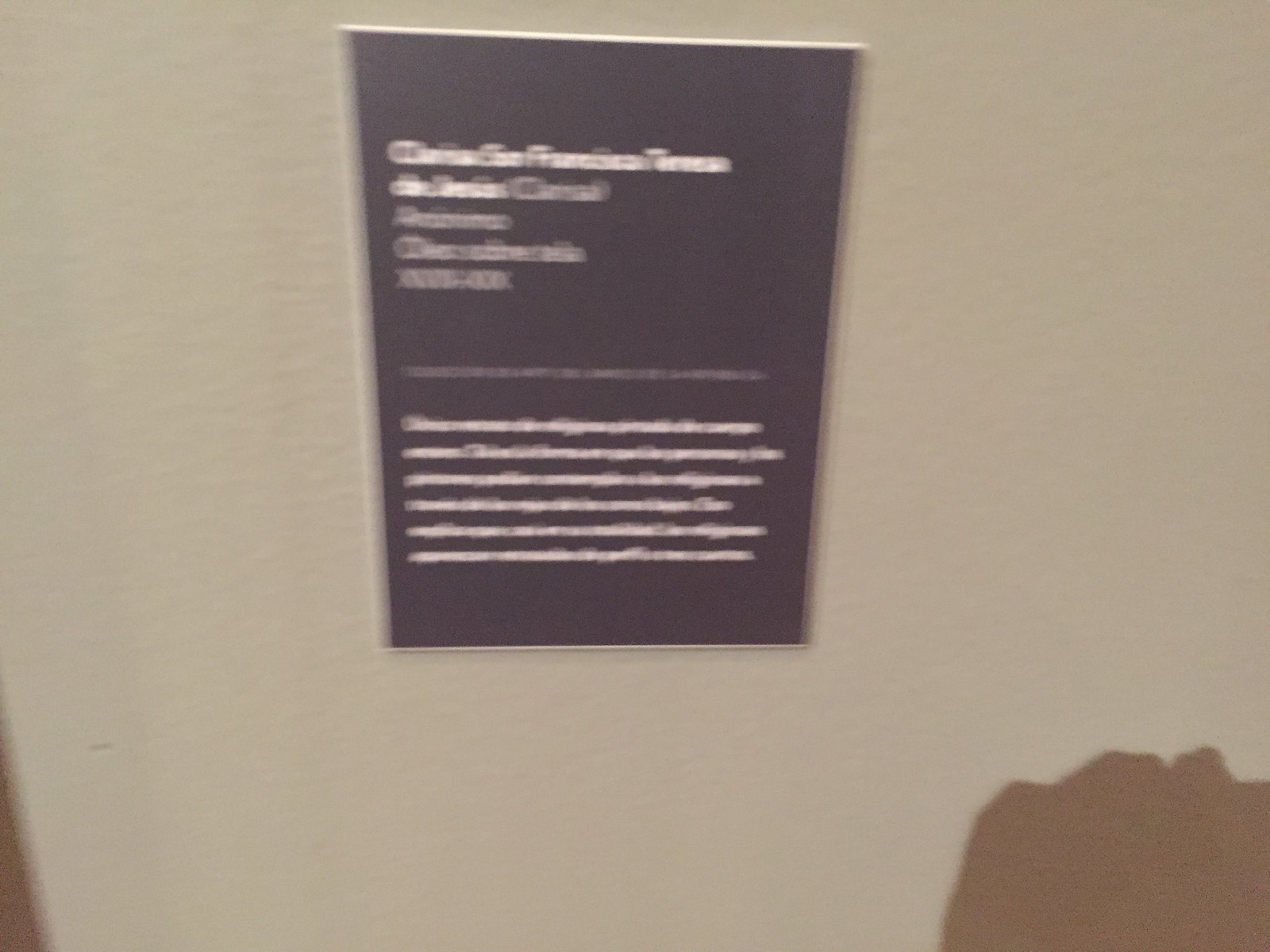This is a colour photograph of a white, textured wall with visible dents and raised bumps. The image is quite blurry and of low resolution, making it difficult to discern details. In the bottom right corner, a thin triangular sliver of brownish color and a dark black shadow can be seen, suggesting areas where the wall might be unpainted or shadows cast by an object. Towards the left, there is a glimpse of brown trim slightly peeking into the image.

At the center top of the photo, there is a black sign with a white rim. Despite its blurry appearance, the sign features white text organized in three sections: bold white text at the top, a lighter white text in the middle, possibly followed by a space, and more white text at the bottom. The text appears to run into each other, making it hard to read, but there are inklings that the language may be Italian or Spanish, with potential words like "San Francisco" and "Franciscan" visible. This could be a doctor's office, hospital, or museum placard, possibly providing informational content or directions within the building.